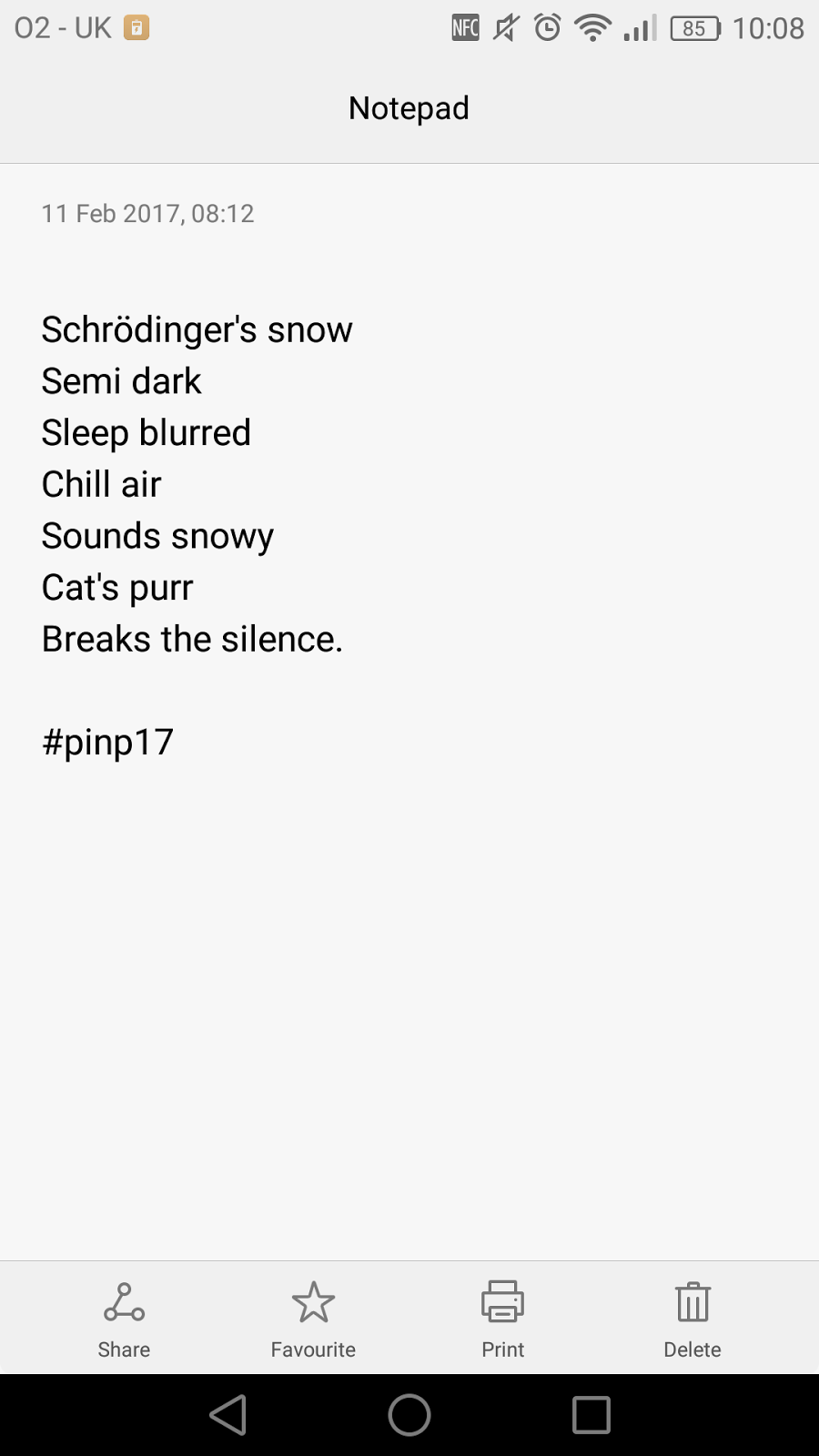Below is a cleaned-up and detailed caption for the described image:

---

This screenshot showcases a smartphone interface against a gray background. The top bar displays the time as 10:08, the date as 11 February 2017, and the battery at 85%. Additionally, there's a 02 UK alarm clock icon. 

The central focus of the screen is a notepad entry that reads:
"Schrödinger's semi-dark, sleep-blurred, chill air. Sounds snowy. A cat's purr breaks the silence. #PINP17"

At the bottom of the screen are several function icons. From left to right, they include:
1. A share symbol.
2. An icon with three interconnected circles forming a triangular pattern.
3. A favorite symbol represented by a star.
4. A print symbol depicted as a printer.
5. A delete symbol shown as a trash can.

Moreover, a black navigation bar at the very bottom features:
1. A triangle pointing left.
2. A circle.
3. A square.

This detailed layout captures the essence of the notepad entry and the array of functional icons available on the device.